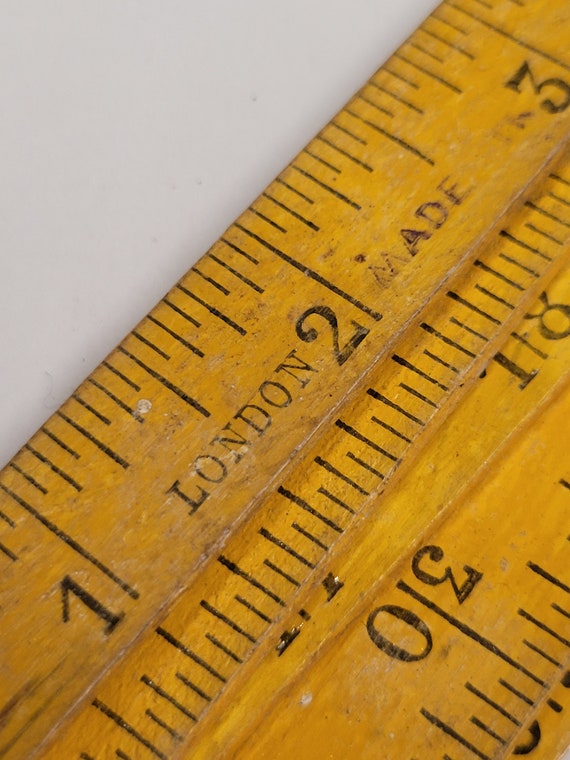This photograph is a detailed close-up view of overlapping wooden rulers, prominently featuring a mustard-yellow ruler at the forefront. The rulers are stacked at an angle, running from the lower left-hand side diagonally to the upper right-hand side of the image. The mustard-yellow ruler shows the inches side, spanning from the 1-inch mark through the 3-inch mark before the ruler extends out of frame. The text ‘London Made’ is present between the 1-inch and 3-inch marks, with the ‘M’ in ‘Made’ notably faded from extensive use. Below this ruler, two other rulers are visible, also wooden and marked, with the bottom ruler clearly showing the number 30 on the centimeters side. The stacked rulers form a composition that creates a dark gray triangular background in the top right center of the image. Despite their overlapping and somewhat uneven alignment, the detailed markings and text on the rulers highlight their well-worn and functional history.